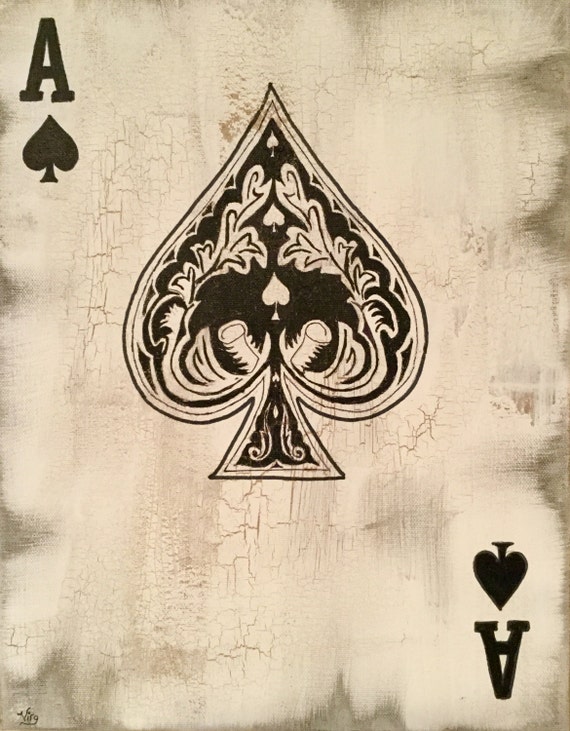This image captures an aged ace of spades playing card in a vertical close-up view. The card, rectangular like a traditional playing card, features an off-white background with evident signs of wear, such as numerous wrinkles, cracks, and a darker tan around the edges, giving it a thoroughly aged appearance. Central to the design is a large, intricately detailed spade symbol, rendered in black with ornate patterns that include smaller spades, leaves, and floral elements. The top left and bottom right corners each bear the black capital letter "A" alongside spade logos. The card also exhibits a more faded and cracked surface with grayish discoloration in some areas, enhancing its vintage look. Notably, there is a signature in the bottom left corner, appearing to say "Virg," suggesting it may have been personally crafted or decorated long ago. The overall black-and-white aesthetic underscores the card's old-school charm and beat-up condition, resembling both an intentionally crafted antique or a naturally aged piece.